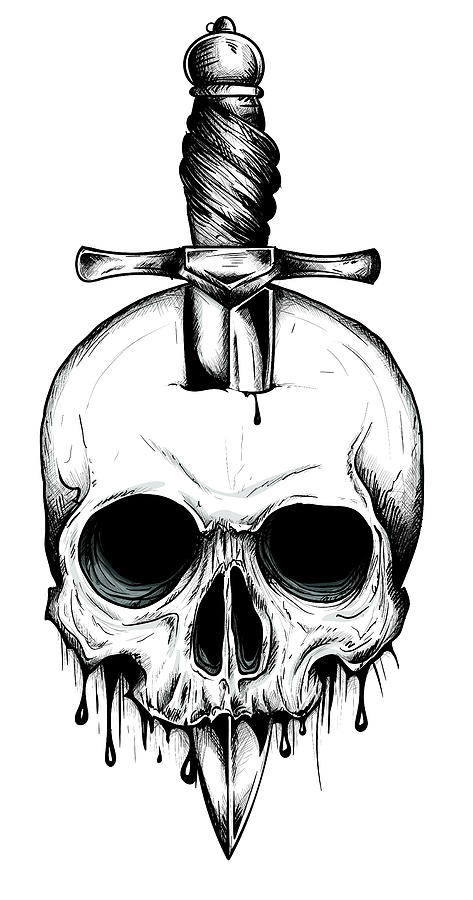This detailed black and white drawing depicts a skull with prominent, hollow eye sockets and a long, dark nasal cavity, accentuated by light gray shading. Notably, a dagger with a cross-shaped handle, adorned with what appears to be twisted rope or fabric, pierces through the top of the skull. The dagger's blade exits through the mouth area, with its pointed tip extending several inches below. The drawing is further intensified by droplets of dark liquid, resembling blood, dripping from the jawless lower part of the skull. Additional drops seem to emerge from a small hole in the forehead, adding to the eerie and somewhat disturbing nature of the sketch. The entire composition, set against a stark white background, conveys an intense and unsettling visual.